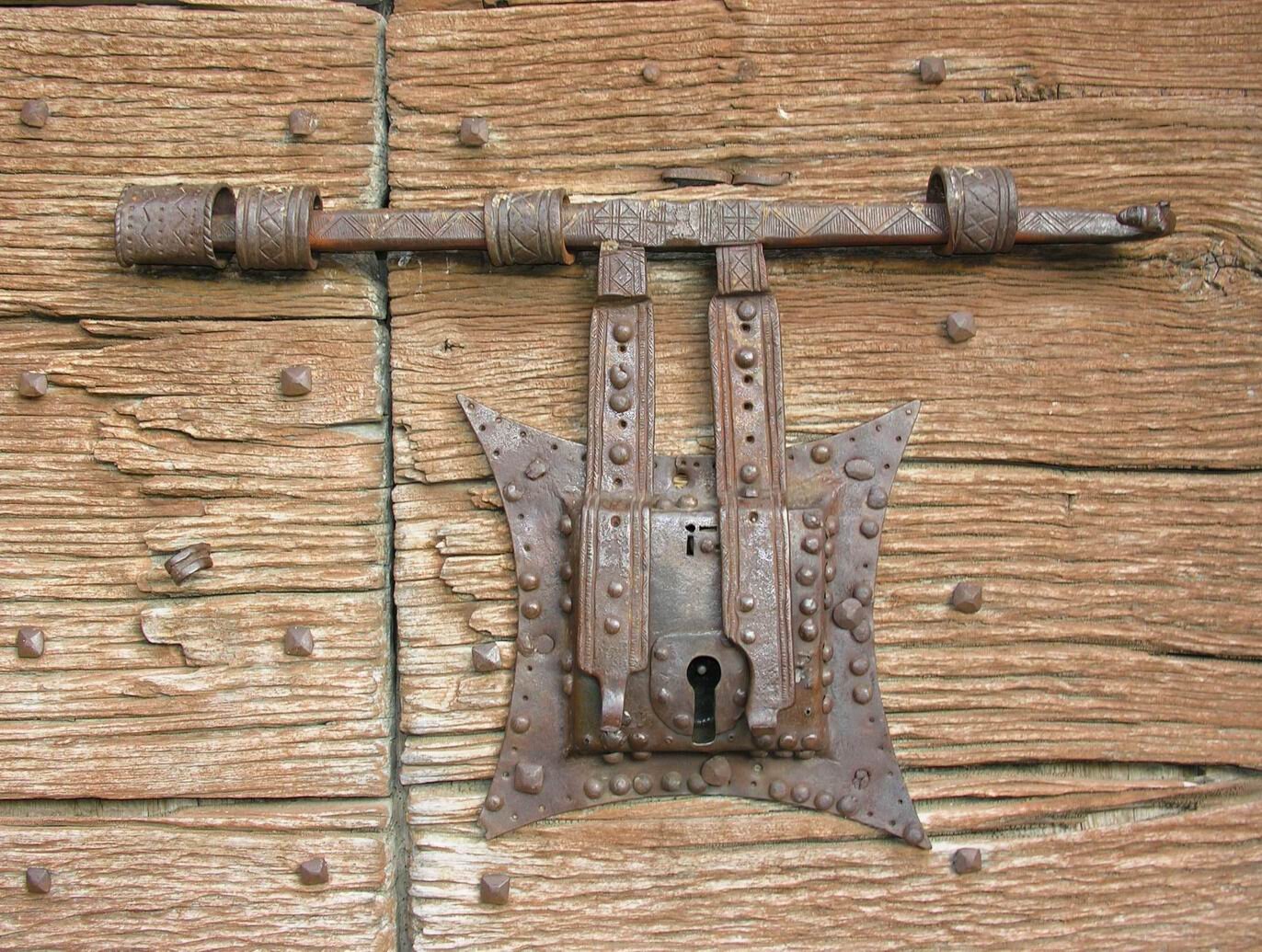This close-up landscape photograph captures an intricately designed, very old lock mounted on ancient, splintering wooden slats. The centerpiece of the image, the lock, appears to be from the medieval ages, boasting a weathered bronze appearance with a T shape. The horizontal locking mechanism slides left to right, securing into bronze couplings on the opposite side of the door or gate. The wood around the lock is cracked and heavily worn, showcasing protruding, bowl-shaped, diamond-head nails that further emphasize its age.

The lock assembly is notably complex, featuring ornate details such as zigzag engravings and small, round bubbles, some of which have broken off over time. The keyhole is of the skeleton type, set within a star-shaped plate, characterized by a square center with spiked corners and dotted edging, giving it a formidable appearance. Above the keyhole, two flat vertical bronze pieces extend upwards, connecting to the horizontally placed engraved metal bar. This bar is secured by loops embedded in the wood, indicating the meticulous craftsmanship of an era long past. The slats of wood are vertically aligned, and to the far left, one can observe a seam where the wood panels meet, potentially marking the entryway.